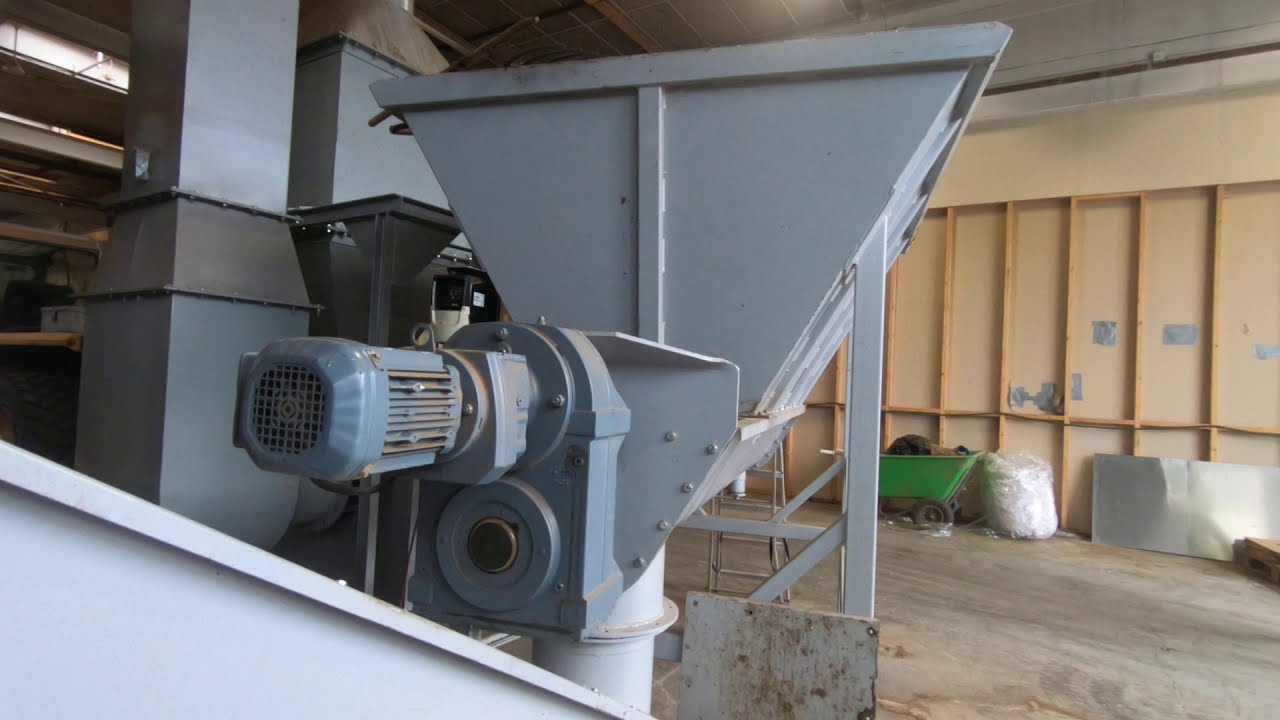The photograph depicts an industrial garage-like setting with a gray concrete floor. Dominating the foreground is a large, gray machine featuring various filters, screws, contraptions, and fans. The machine has an upside-down pyramid shape at the top, with a chute connected to some sort of motorized system and further machinery, which is partially obscured. The machine also sits on a rusted base. To the left side, fluorescent lights illuminate the space, and there are beige walls with visible wooden beams or 2x4 framing.

On the right side, leaning against the wall, is a large piece of sheet metal next to a clear plastic bag filled with what appears to be shredded material or paper. In front of this, there is a green wheelbarrow containing unidentified items. Further toward the back, the space becomes darker but hints at a metal gray box, adding to the industrial ambiance.